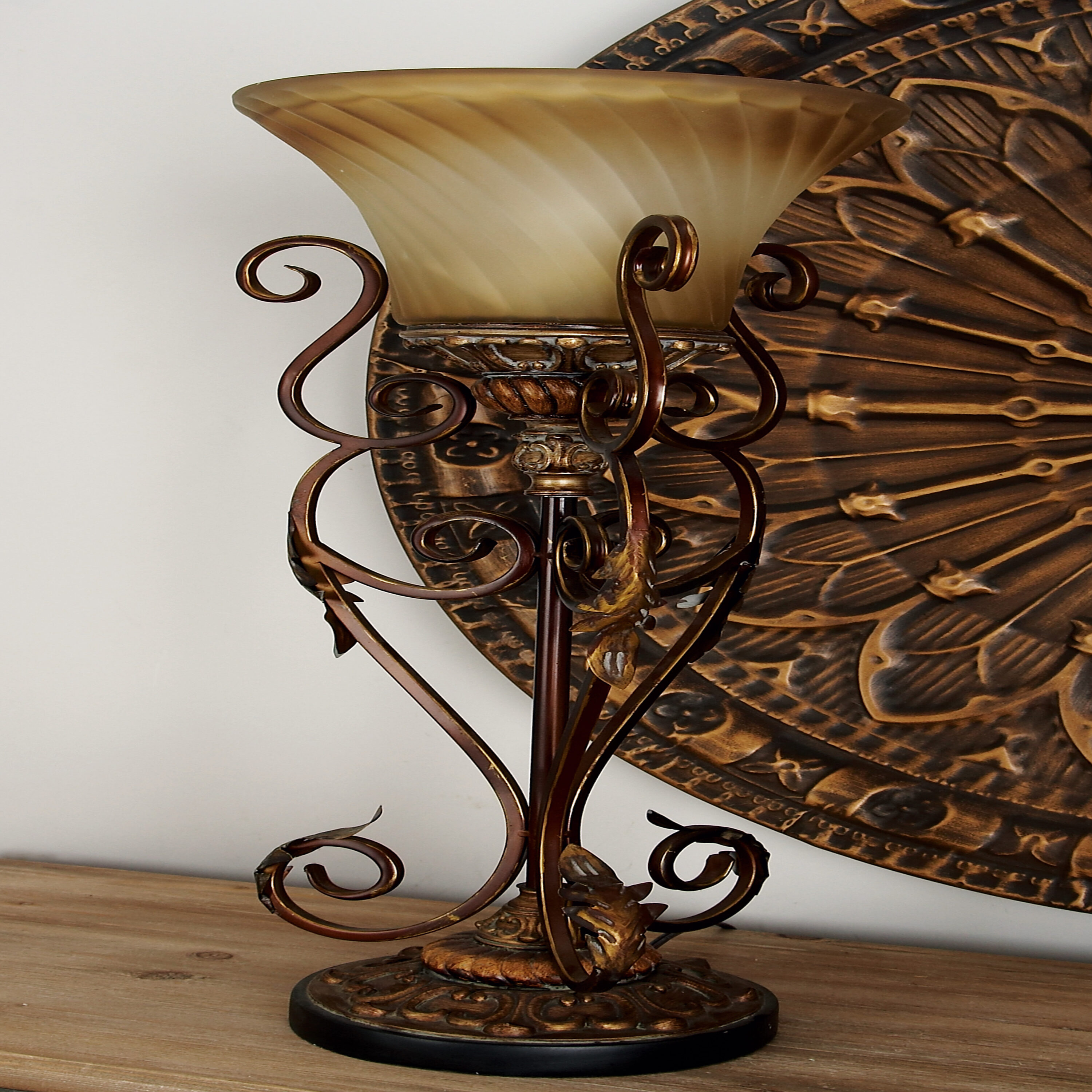The image showcases an intricately designed lamp with an antique or vintage appearance, possibly a reproduction of an older style. The lamp features a substantial bronze base with dark, intricate curled metalwork patterns, and three bent metal rods that curl elegantly upward. Atop the rods is a flaring, beige glass cover that functions much like a torch, dispersing light outward rather than downward. Behind the lamp, attached to the white wall, is a bronze circular plate adorned with star-shaped cutouts. The lamp, along with this decorative wall piece, rests on a narrow, wooden table or shelf. The overall setting is minimalistic, with the focus primarily on the lamp’s elaborate and artistic metal and glass craftsmanship.